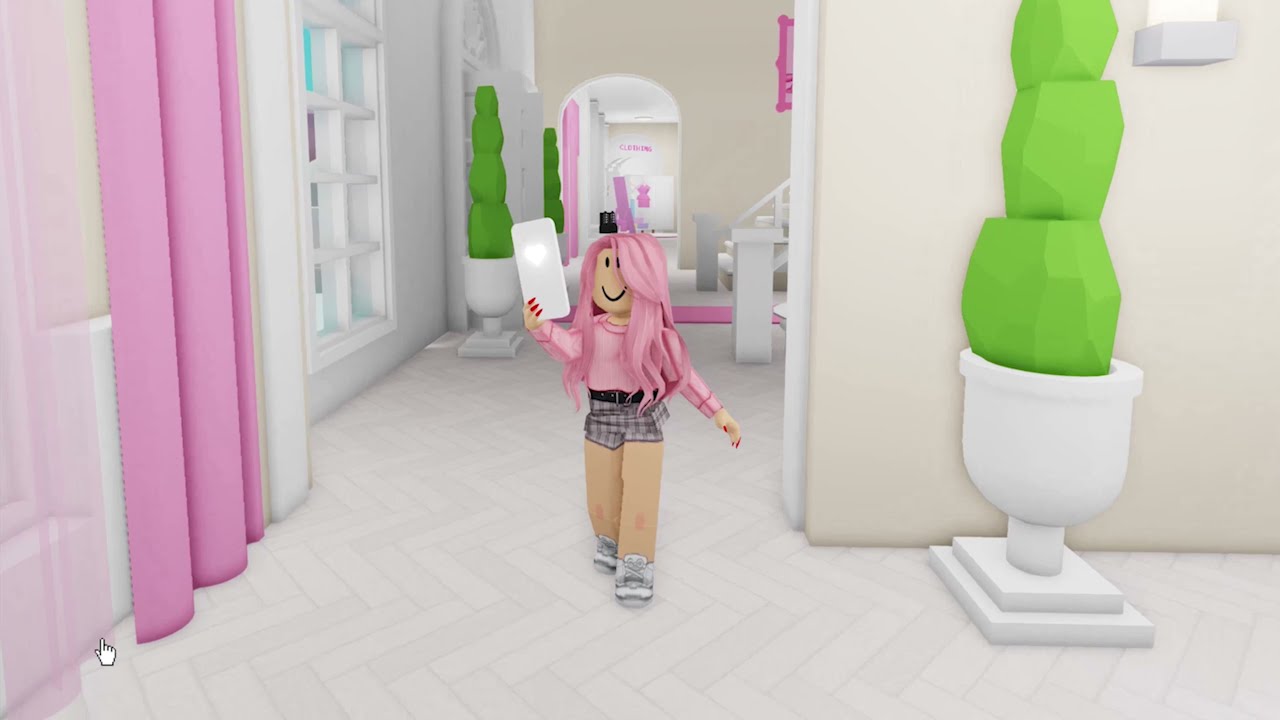The image depicts a detailed and imaginative scene that combines elements of reality and whimsical design. At the center is a cartoonish, cardboard cutout of a girl with a smiling face, characterized by long pink hair, oversized red fingernails, and a pink long-sleeve sweater that ends at her waist. She is dressed in gray shorts and gray sneakers, and her top in this instance aligns more with a pink shirt. The girl holds up a very large white cell phone or tablet—almost the size of her body—featuring a heart on its back, appearing as though she is taking a picture or deeply engrossed in it. Her simplistic facial features include two dots for eyes and a curved smile.

The backdrop showcases an entrance area of a large, blocky house adorned with various green plants. On the right, there is a three-tiered shrub placed in a white planter that looks similar to three round balls of Play-Doh stacked together. Further left, there is a hallway where two more identical four-tiered bushes in white planters are visible. The setting denotes an artistic touch, likely resembling cardboard or paper mache, painted to appear realistic with pink curtains that drape down to the white floors from a white window with eight square panes. The scene emanates a playful yet surreal atmosphere, blending tangible household elements with a cartoon-like aesthetic.